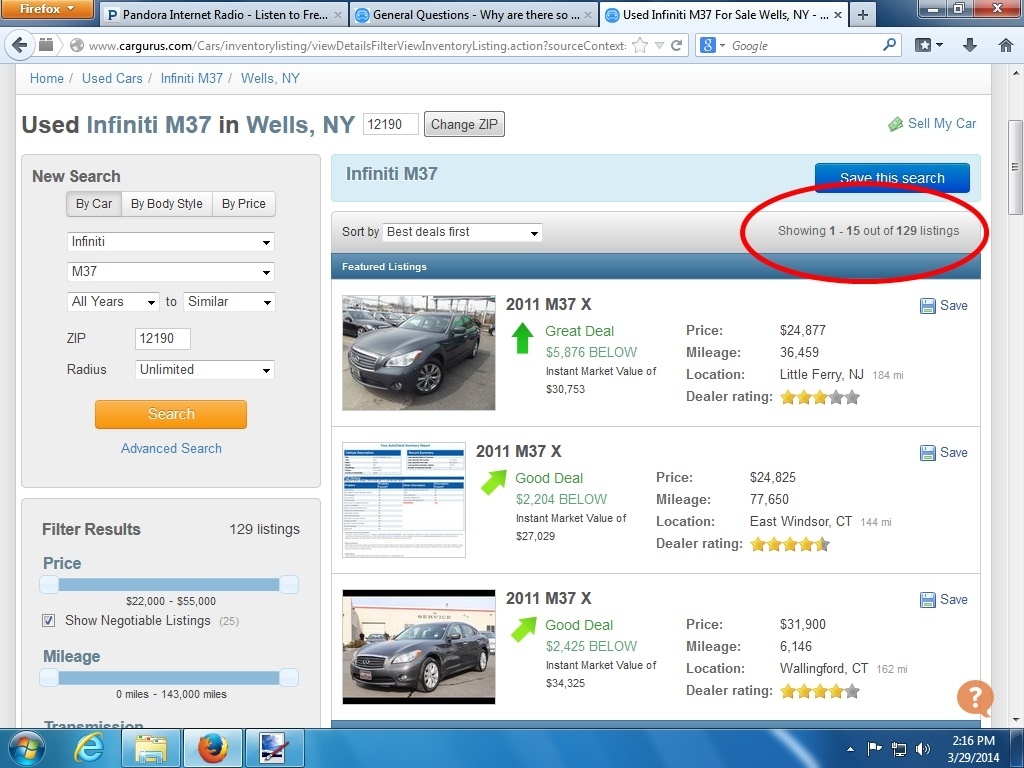This is a detailed screenshot of a Firefox web browser window. At the top, the browser's header indicates "Firefox" next to an orange drop-down menu with white font. To the right of the header, three tabs are open. The first tab is titled "Pandora Internet Radio, listen to fre..." The second tab reads "General Questions - Why are there so..." The active tab is titled "Used Infiniti M37 for Sale, Wells, New York." 

To the far right of the tabs, the minimize, maximize, and close buttons for the web browser are visible. Below the header, a search field shows the URL "www.cargurus.com." The main content area of the webpage displays a search interface for used cars. At the top left, a blue navigation path reads "Home / Used Cars / Infiniti M37 / Wells, New York." Beneath this, in grey font, it says "Used Infiniti M37 in Wells, New York, 12190" with an option to "change zip." Below this heading, the search results show "1 out of 15 of 129 listings," indicating a summary of available Infiniti M37 listings in the specified location.